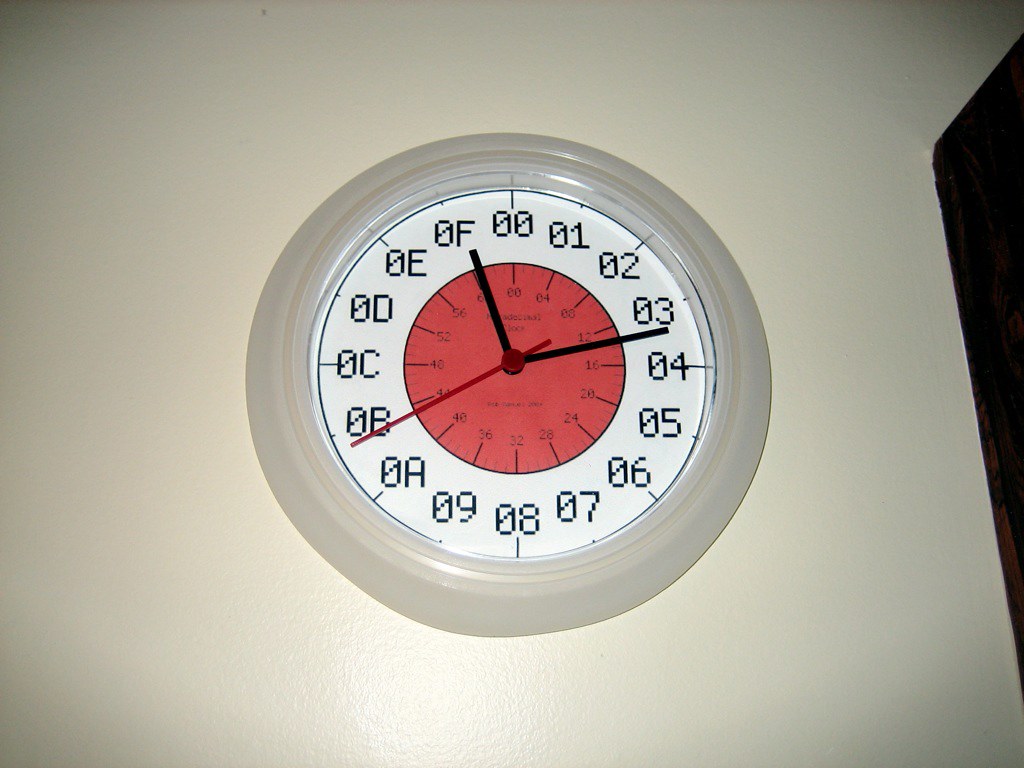The image features a unique clock, prominently displayed against a plain white wall, centered within the frame. The clock has a strikingly thick white border, likely made of plastic, which encases its predominantly white face. At the center of the clock face, a vivid red circle draws attention.

The clock possesses three hands: two of which are black, and a distinctive third hand that is red. Unconventionally, the numbering on this clock deviates from the traditional 1 through 12. Instead, the numbers range from 0 to 8 and then transition into letters.

Starting from the top center and moving clockwise along the outer rim, the sequence is peculiar: 00, 01, 02, 03, 04, 05, 06, 07, 08, followed by 09, and then letters 0A, 0B, 0C, 0D, 0E, and 0F, before looping back to 00. Within the center red circle, there is another series of smaller, less legible numbers that appear to increase in multiples of 4.

This clock’s numbering system, involving both numbers and letters, and the additional inner circle of numbers, suggest it is not a conventional timepiece. Its purpose remains ambiguous, though the intricate detail implies a specialized function possibly related to a particular field or form of measurement.